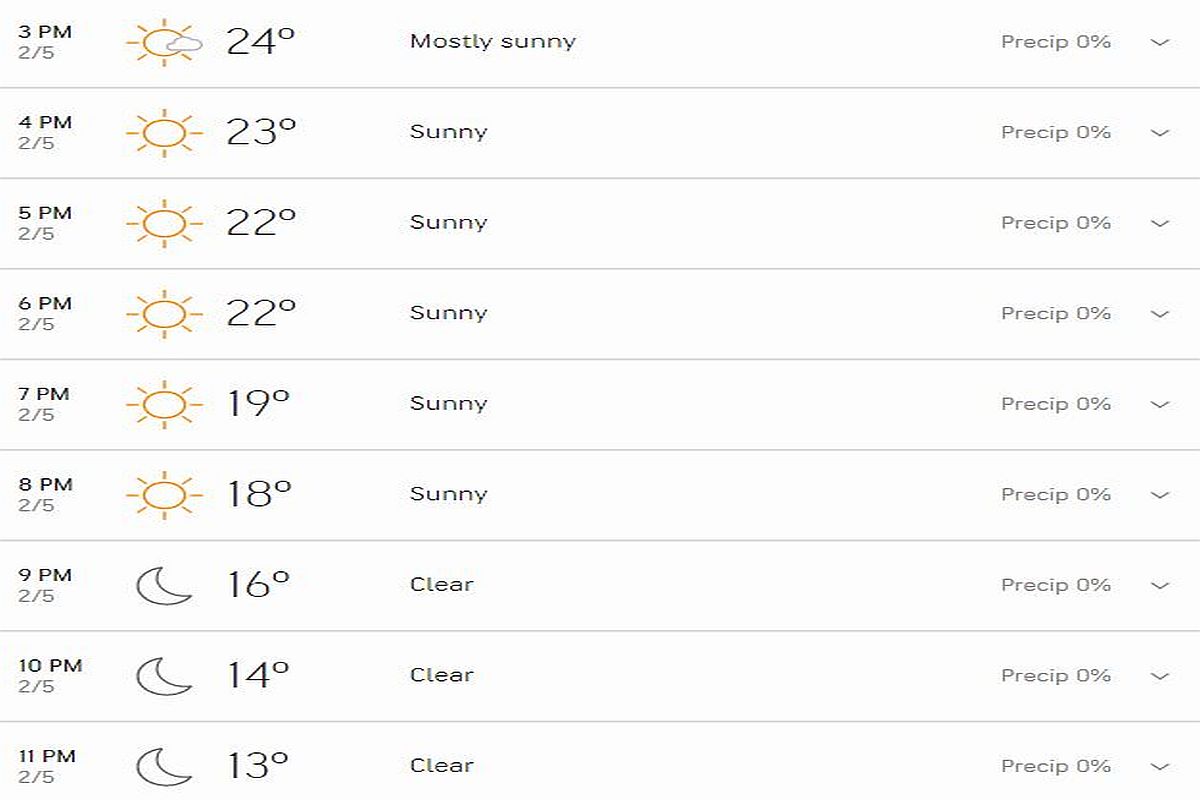The image depicts a smartphone screen displaying a detailed hourly weather forecast. On the left side of the screen, times are listed starting from 3:00 PM on February 5th. Adjacent to each time slot is a weather graphic indicating the conditions for that hour, followed by the temperature and a description of the weather. On the far right, precipitation probabilities are noted.

At the top, for 3:00 PM, the forecast shows partly sunny weather represented by an icon of the sun partially obscured by a cloud, with a temperature of 24 degrees and 0% precipitation. From 4:00 PM to 8:00 PM, the condition changes to sunny, with the temperature gradually decreasing from 23 degrees to 18 degrees. At 9:00 PM, the icon shifts to a moon, indicating clear skies and a temperature of 16 degrees. The clear weather continues through 10:00 PM and 11:00 PM, with temperatures dropping to 14 degrees and then 13 degrees respectively.